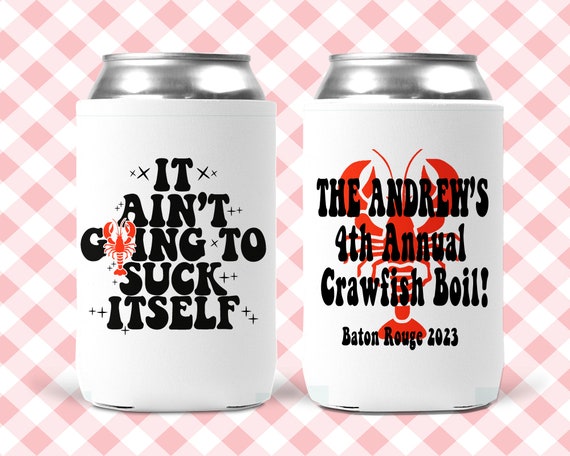This image showcases an ad poster for Andrew's 9th Annual Crawfish Boil in Baton Rouge, 2023. The poster features two shiny silver beer cans prominently displayed against a light pink and white, pastel checkered background reminiscent of a picnic tablecloth. The cans are wrapped in white koozies, each adorned with different text and graphics. The can on the left displays the phrase "It ain't going to suck itself," with a stylized red lobster in place of the "O" in the word "going." The can on the right features a red lobster logo, accompanied by the text "Andrew's 9th Annual Crawfish Boil" in black font. The background includes an illustrated red lobster, enhancing the festive and playful theme of the advertisement for the event.